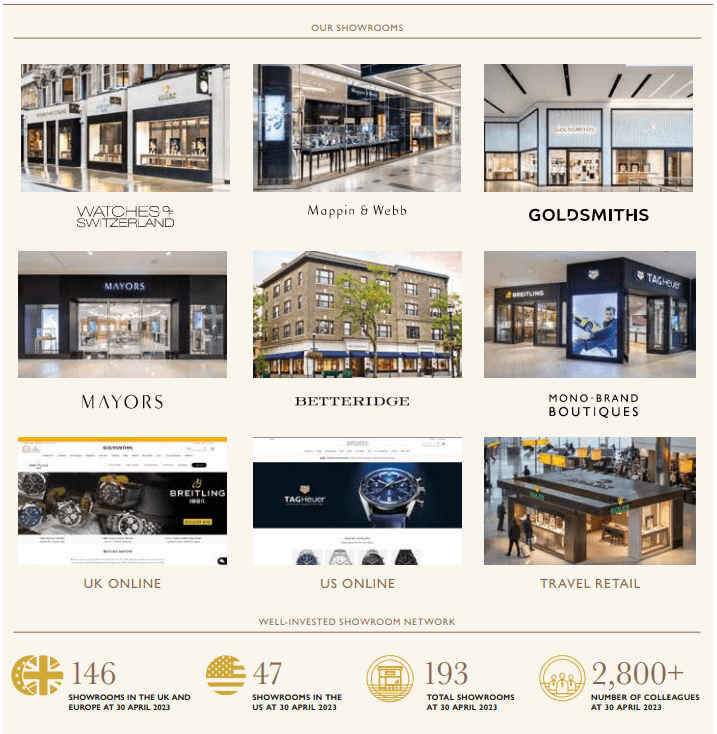This image captures a wide array of luxurious showrooms belonging to Watches of Switzerland Group, including esteemed brands such as Goldsmiths, Mayors, and Betteridge, as well as various Monobrand boutiques. It highlights their expansive presence with detailed mapping of both UK and US locations. Specifically, the image represents a total of 193 showrooms across both regions, with 146 showrooms situated in the UK and Europe and 47 in the US, all as of 30 April 2023. Additionally, the visual indicates the company's substantial workforce, comprising over 2,800 colleagues as of the same date. The bustling environments of the showrooms and the architectural elegance of the buildings are prominently featured, portraying the opulence and widespread reach of the Watches of Switzerland Group in both physical retail and online platforms.